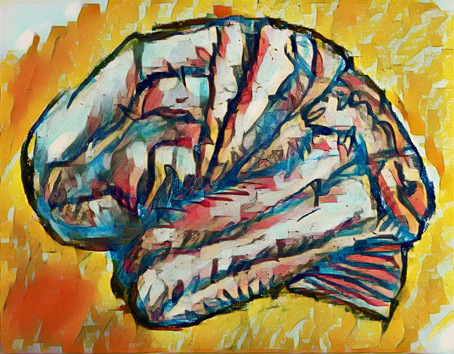This artistic rendering, likely created with watercolors, presents a vibrant and abstract depiction, potentially symbolizing a human brain, a turban, or a seashell — interpretations vary. The central object, whose shape suggests creases and folds akin to textiles or organic forms, is intricately detailed with numerous hues, including white, various shades of blue, red, orange, black, brown, tan, pink, and touches of green. These colors blend seamlessly into one another, enhancing the abstract nature of the image. Surrounding this central figure is an expressive background dominated by energetic strokes of yellow and orange, interspersed with patches of white and light blue, particularly concentrated in the upper right and corners. The overall texture and style, characterized by its scribble-like patterns and black outlines, reinforce the dynamic and evocative quality of the artwork, making it a striking piece whether viewed as a brain, a turban, or a seashell.